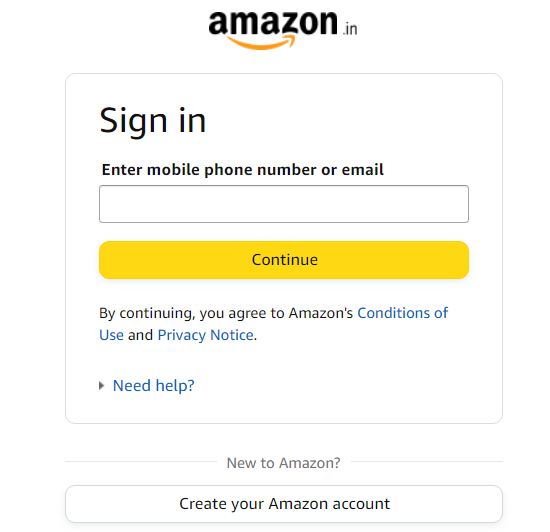The image showcases a login screen for Amazon's Indian website, denoted by the ".in" domain. At the top, the iconic Amazon logo is displayed in bold black lowercase letters, featuring an orange arrow that extends from the first "a" to the "z," symbolizing Amazon's extensive range of products from A to Z.

Below the logo, the main section of the login interface is encased in a white rectangle with a gray border. The first line of text prompts users to "Sign-In" in bold black letters. Directly beneath this, another prompt states "Enter mobile phone number or email," indicating the required input with each word beginning in uppercase.

A white text box outlined in black follows, allowing users to type in their contact details or email address. Positioned below the text box is a yellow rectangular button with the word "Continue" centered in black uppercase letters.

Further down the interface, a brief message reads: "By continuing, you agree to Amazon's Conditions of Use and Privacy Notice," where "Conditions" and "Privacy Notice" are highlighted in blue, making them look like clickable links.

Finally, at the bottom right corner, a gray arrow points to the phrase "Need help?" in blue lettering. This is followed by a gray prompt asking if the user is "New to Amazon?" and ends with an invitation in black text, "Create your Amazon account," suggesting that new users can easily register for an account.